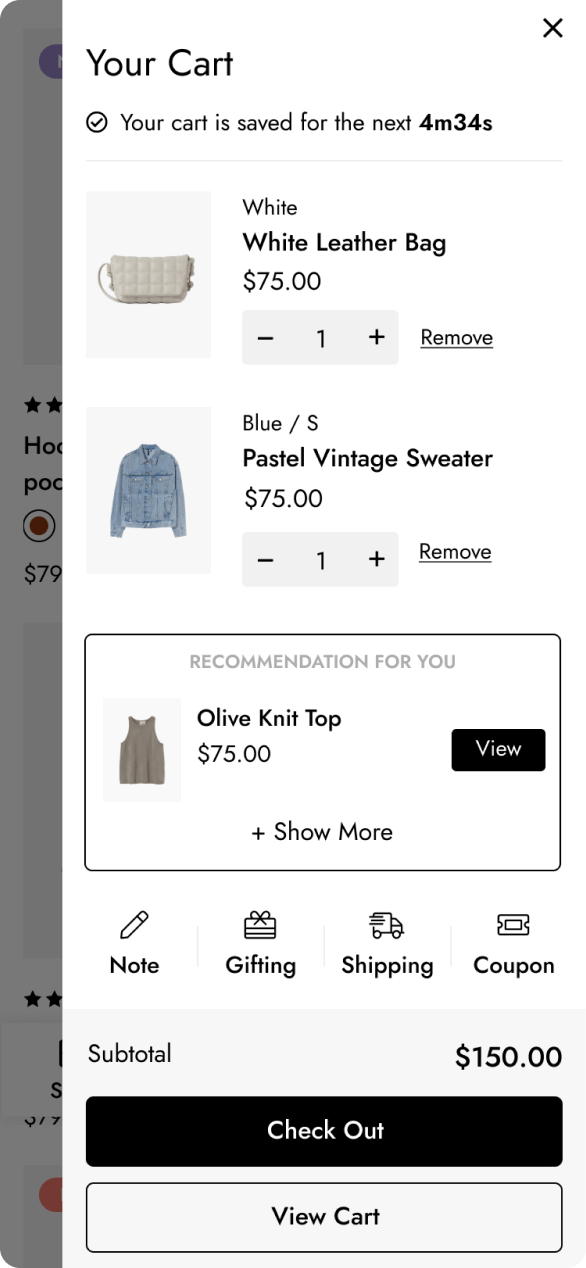You are viewing your shopping cart on a retail website. Your cart will be saved for the next 4 minutes and 34 seconds. Inside your cart, there is a small, white leather bag with a quilted, padded design, retailing for $75. Additionally, you have a small, pastel blue vintage sweater, also priced at $75. There is also a recommendation for an olive knit top at the same price, $75, with the option to view more like it.

So far, your total is $150 for the white leather bag and the blue vintage sweater. You have the option to proceed to checkout or continue browsing the cart. Options are available to add a note, choose gift wrapping, specify shipping details, or apply a coupon.

If you decide to close the cart, you can explore the website further, where items start at around $79 and come in various colors. But for now, you have just under five minutes to finalize the purchase of the white leather bag and the blue vintage sweater, or explore the recommendation for the olive knit top before making your decision.